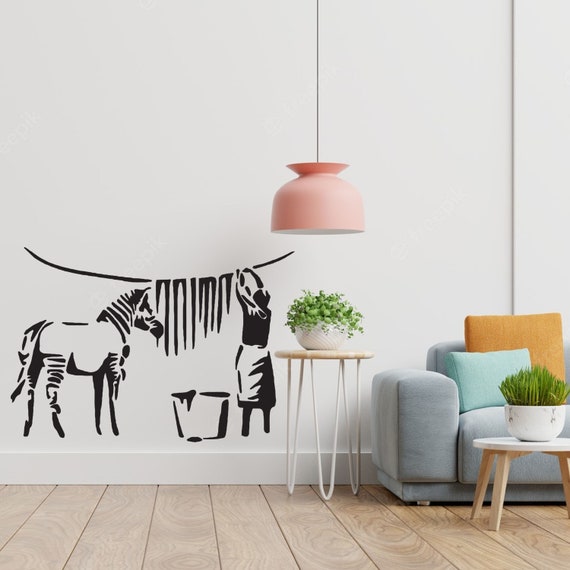This photograph features a contemporary living room with light wooden hardwood floors. Dominating the space is a white wall adorned with a unique black mural depicting a zebra missing some of its stripes, which are hanging on a clothesline with the help of a woman in a skirt and apron. Suspended from the ceiling is a pink dome-shaped lamp, casting light over a potted plant positioned on a white-legged stand. To the right, a grayish-blue sofa partially appears, showcasing two pillows—one large and orange, the other smaller and light blue. A coffee table with a white surface and light wooden legs stands in front of the sofa, holding another plant in a white bowl. The minimalist yet artistic setting conveys a blend of functionality and creative decor.